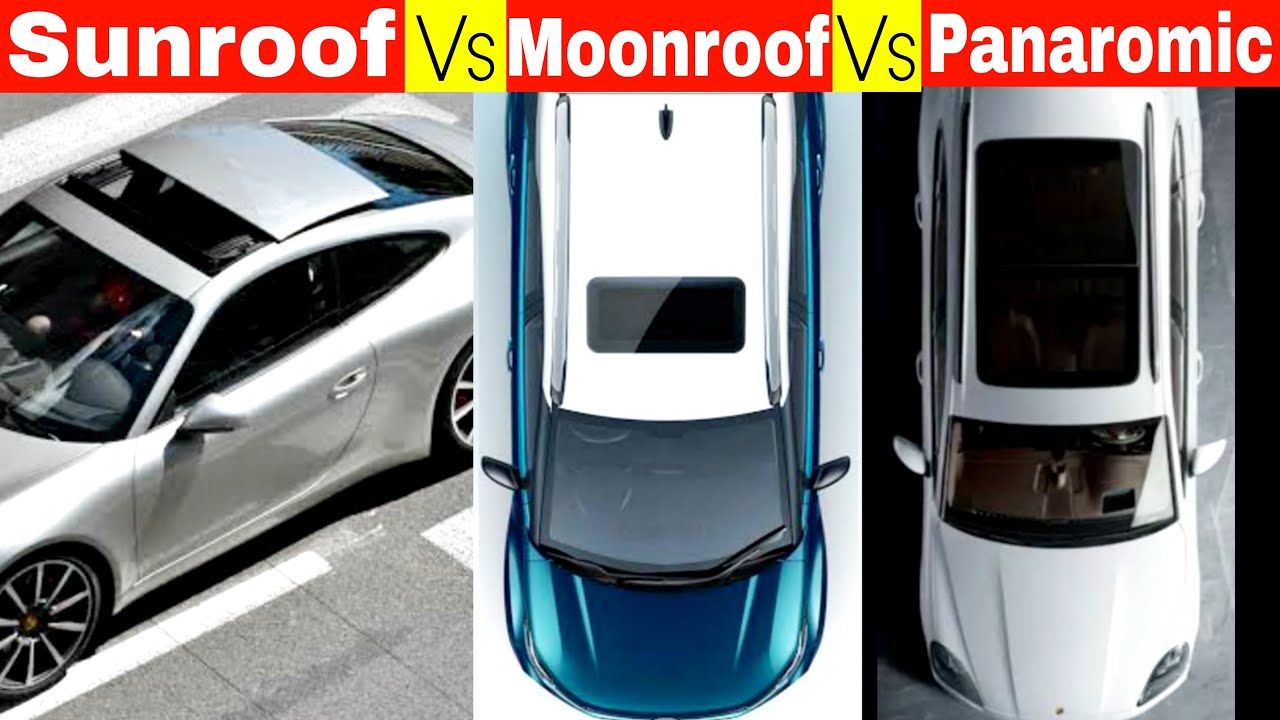This image showcases a top-down view of three cars, each illustrating different types of roof windows. The comparison highlights three roof styles: sunroof, moonroof, and panoramic, with labels in white text on red backgrounds at the top of each segment. Between these labels, yellow boxes with black "VS" lettering indicate the comparisons. 

The car on the left features a standard sunroof, which appears to be an automatic, retractable panel allowing open sky access. The middle car displays a moonroof, characterized by a smaller, fixed glass panel that might have an interior slide shade but doesn't open. The car on the right exhibits a panoramic roof, an expansive glass panel spanning the length of the roof from front to back, providing a full overhead view. Each car is oriented with the front at the bottom of the image and the rear at the top, positioned on a sidewalk.